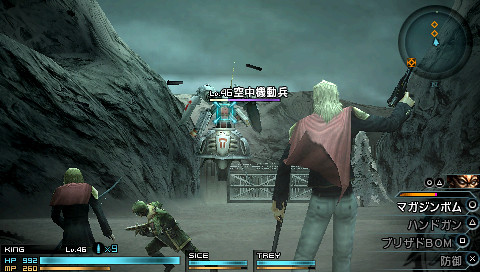The image is a highly detailed screenshot from a Japanese video game. The main character, viewed from behind, stands center stage amidst a dynamic scene set in a rocky valley. This character, who has long white hair, wears gray pants with two back pockets and a rust-colored long-sleeve shirt. Draped over his shoulders is a pink shawl or cape with a darker underside, flipped to the left. His posture shows his left arm pointing straight down while his right arm is bent at the shoulder, holding a gun with an orange symbol at its barrel. Surrounding this character are other figures: one to the right with green hair and jeans, also seen from the back and sporting a red cape, and two others to the left, seemingly preparing for battle. These other characters also hold weapons, indicating readiness for combat.

A large, flying machine is seen approaching the characters, suggesting an imminent confrontation. At the bottom of the screen, various game HUD elements are visible, including a turquoise HP bar displaying "HP 992," an orange bar indicating "260," and labels showing "King level 46." Japanese characters are present in multiple areas, such as the bottom right and mid-screen, lending context to the game's interface. The setting, characters, and graphics all point towards a climactic battle, likely against a significant boss monster, hinted at by its health bar and foreign script above it.